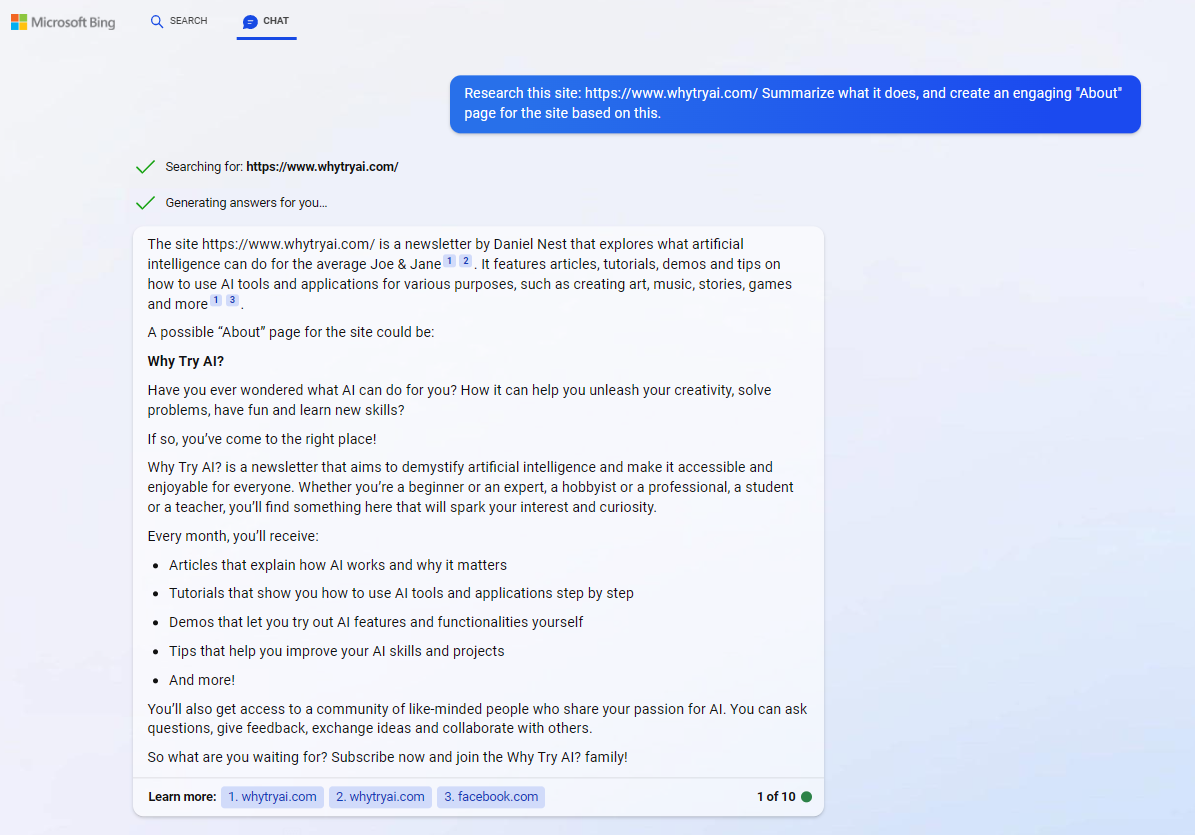This screenshot showcases a digital interface with distinct blue and white chat boxes. The blue chat bubble contains the text "Why try all," while the white chat box includes several pieces of fragmented text such as "one of 18," "learn more," and "Microsoft," located in the top left corner. Additional text within the interface includes "enter," "search the site," "summary," "what," "dies," and "create a mapping about page for the she based on bills."

The webpage appears to be a research-oriented site dedicated to exploring artificial intelligence and its alignment with everyday individuals, indicated by the phrase "site is a research to deny meat that explores while artificial alignment for to the average Joe and me now." This caption encapsulates key screen elements and the overall theme centered around AI research.